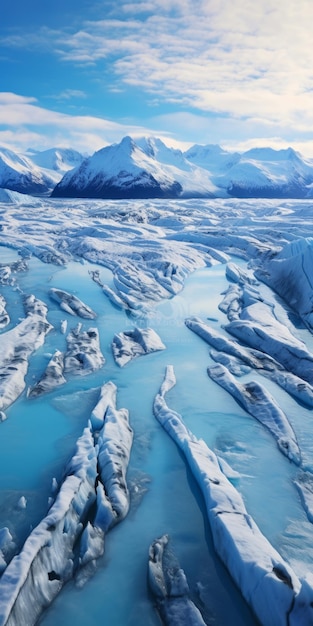The photograph showcases a breathtaking Arctic landscape dominated by snow-covered mountains, with a central peak surrounded by several others of similar height. The top third of the image features a vivid blue sky adorned with faint white clouds, creating a picturesque backdrop. Below the mountains lies a beautiful, light blue waterway, partially frozen and interspersed with icy formations and glacier segments. The scene is predominantly white and blue, with the reflective water mirroring the sky's hues. The overall composition of snow, ice, and water, along with the sculptural ice formations in the foreground, creates a striking and serene Arctic vista.